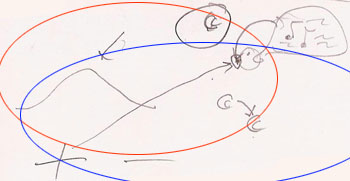The image is a children's drawing on a white piece of paper, characterized by its messy and scribbly appearance. Prominently, there is a large, perfectly drawn red circle, which suggests it was traced. Adjacent to it is an even larger blue circle, somewhat oval in shape, with part of it cut off at the edge of the paper, and this too appears to be traced.

Amidst the scribbles in black pen, several intriguing elements emerge. Two distinct X marks are visible, alongside a series of erratic lines. One particular feature stands out: a stick figure with a notable face at the end of a long line, possessing a single dot for an eye and an open mouth, indicative of singing. Accompanying this depiction are musical notes encased within a circle, suggesting the expression of music.

Additionally, another circle is present featuring a "C" shape, whose significance is unclear. Within this circle, there are additional "C" shapes, an arrow, and other marks which might relate to the musical theme conveyed by the stick figure.

The drawing's chaotic and unrefined style strongly indicates that it was created by a young child, adding a layer of charm to this imaginative artwork.